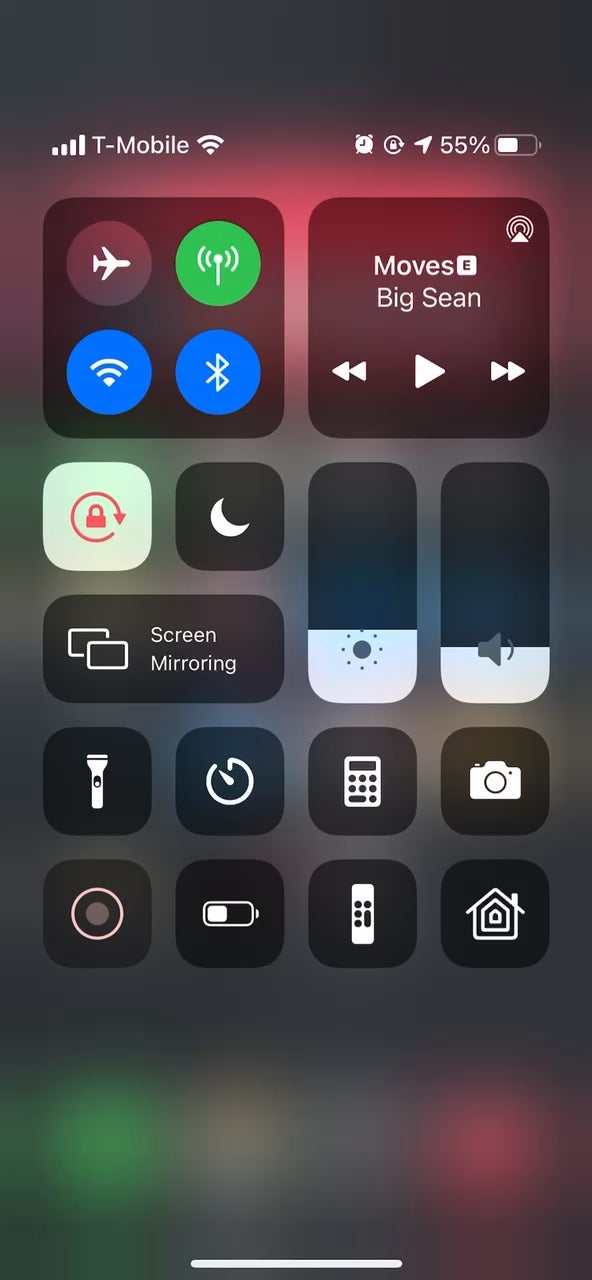The image features a gradient background transitioning from black at the top to dark gray at the bottom. The background includes blurry elements, creating a misty effect. A semi-transparent gray menu overlays this backdrop, adding to the complexity of the image. A purple haze is visible near the top section, while vibrant green, white, blue, and red lights streak horizontally across the bottom.

In the top left corner, four signal bars indicate a full T-Mobile connection, accompanied by a full Wi-Fi signal icon. The top right corner displays an alarm clock icon, a message notification showing "55%", and a battery icon. Below these, there is a black square with icons for airplane mode, Wi-Fi, Bluetooth, and 5G connectivity.

Adjacent to the square on the right, another section contains text stating "Moved Big Sean" and features media control buttons for back skip, play, and forward skip. Below this section, slightly to the left, there is a white square with a red lock icon and a curved arrow encircling it.